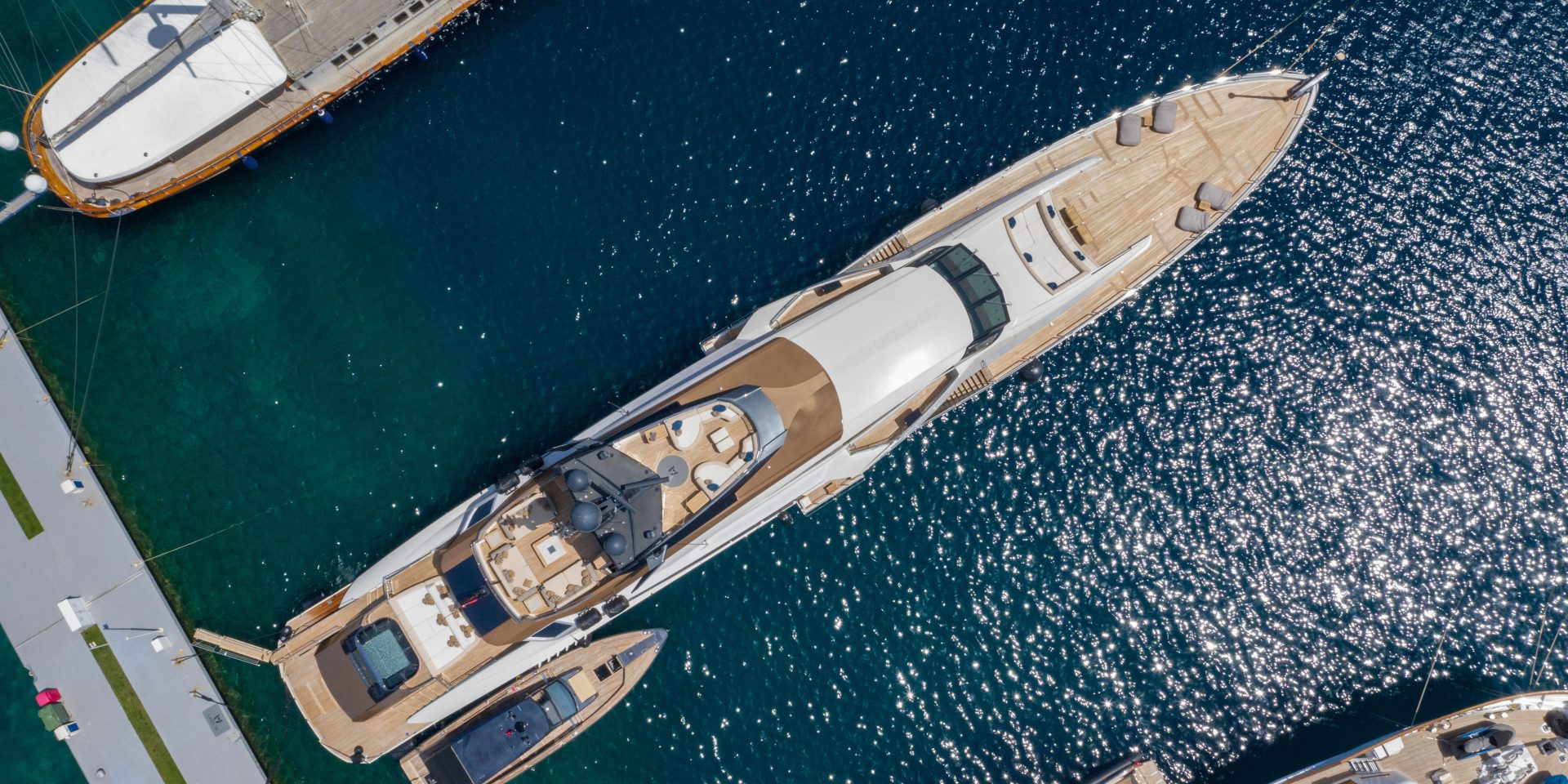The image captures an aerial view of a long, white yacht docked in beautifully sparkling, blue water on a bright, sunny day. The yacht's beige areas, likely wooden deck sections, are where people might gather, including the upper deck with benches and tables. This yacht is the central focus of the horizontal photo, running diagonally from the bottom to the top of the image. We see the hint of another yacht’s corner in the top left, but the main yacht's impressive length dominates the scene. The vessel is flanked by a smaller black and beige boat on its right side, near its aft section. This smaller boat is about one-fifth the length of the yacht and half its width. The dock next to the yacht resembles a narrow gray road. The calm yet slightly rough water beneath glistens with sunlight, adding a serene yet vibrant feel to the photograph.